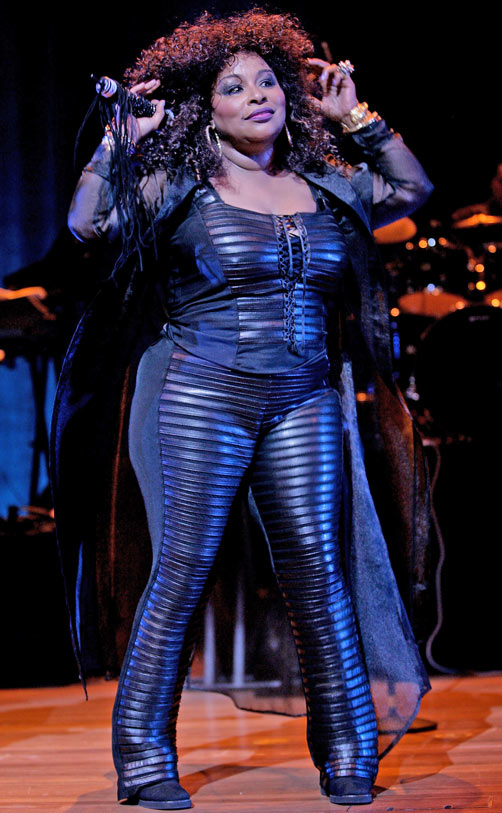In this image, an African American female singer, identified as the famous Chaka Khan, is performing on stage. She is in an all-black, intricately designed rubber suit, accented with a sheer black cape that features red outlines or stitching. Her outfit uniquely combines materials like leather and velvet, rendering it exceptionally artistic and fashionable. Chaka Khan's right hand holds a microphone, while her left hand, adorned with a massive diamond ring and a large gold bracelet, is raised to her temple. She also wears several gold jewelry pieces, including chains or watches, on her left hand. Sporting wild, curly hair styled in a voluminous afro, which appears to have a reddish tint, she exudes an iconic stage presence. Her lips are painted with striking purple lipstick. In the background, dimly lit drums and other musical instruments can be seen, and the hardwood floor of the stage is noticeable. Strobe lights illuminate her, creating a dramatic atmosphere with no text visible in the scene.